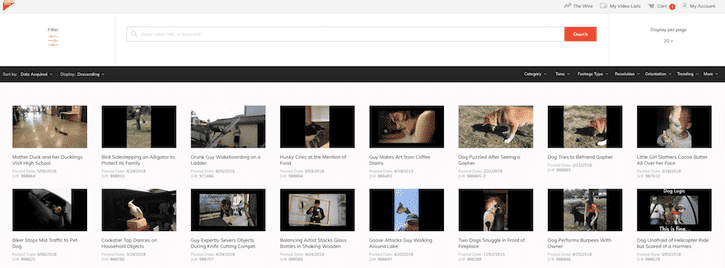This is a detailed caption for the given image:

---

The screenshot is of a webpage, though the small size makes the details challenging to discern. At the top of the page, there is a gray rectangular header. In the upper left corner of the header, there is a red triangular icon, though its details are not clearly visible. On the upper right corner, red text displays navigation options such as "The Wire," "My Video List," "Cart" (indicating one item in the cart), and "My Account."

Directly below the header is a large search bar with a red search button on the right. Beneath the search bar, gray text reads "Display per page: 20+." Following this is a black bar containing various search filters including "Category," "Time," "Format," "Population," "Orientation," "Trending," and "More."

Below the search filters are rows of video thumbnails. There are two lines, each consisting of around ten video thumbnails accompanied by black text descriptions underneath them. One of the videos is titled "Mother Duck and Her Ducklings Visit High School."